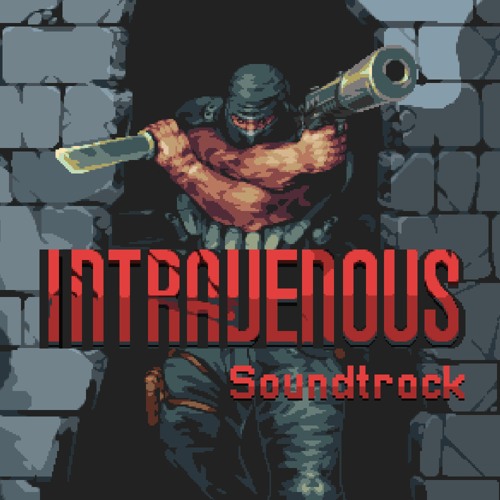This square-shaped image, roughly 3 to 4 inches on each side, appears to be a cover for a retro video game soundtrack titled "Intravenous." The pixelated, low-resolution art evokes the style of old Nintendo games and depicts an intense scene. A towering, muscular man dressed in black tactical gear and a black balaclava with only his eyes visible through a slit, bursts through a broken stone wall. He exudes a menacing presence with his arms crossed in front of his chest, holding a large knife in his left hand and a silenced gun in his right, both pointing opposite directions. The background is a dark entryway framed by stone cinder block walls. The man's outfit, including a holster on his leg and potentially grenades around his midsection, adds to his formidable appearance. Large red text in the center of the image reads "Intravenous," with "Soundtrack" written below it in smaller red text, indicating this cover represents a musical album likely related to a violent animation or game.